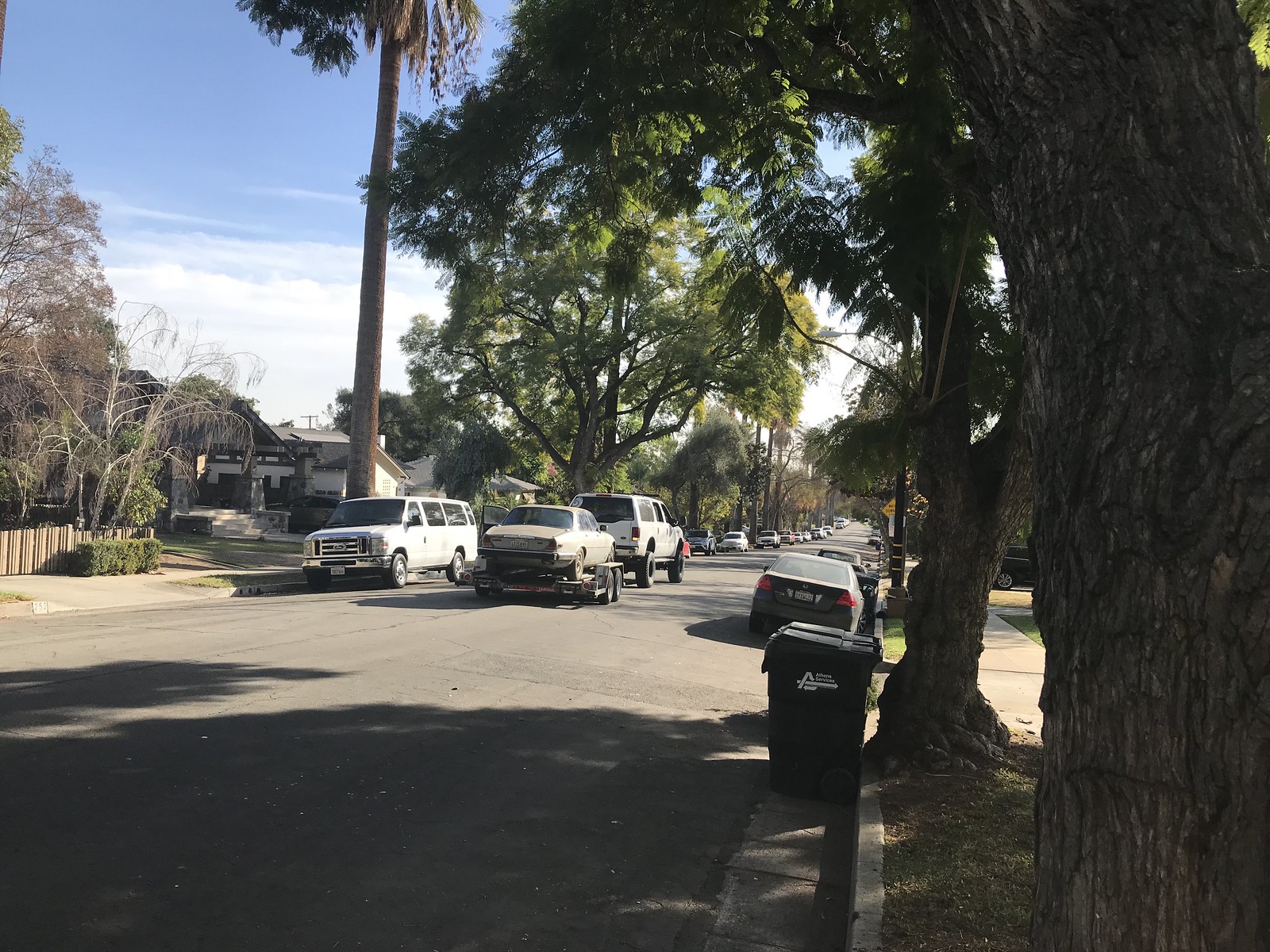A wide street scene bathed in daylight with a picturesque blue sky and fluffy white clouds overhead. On the upper left, a tall tree stands majestically among smaller trees, flanked by a quaint wooden fence with a small bush in front. In the background, several houses peek through, partially obscured by more trees. A tall tree trunk towers above, with a van parked in front of it. The street extends to the right, lined with more trees and parked cars. Down the middle of the road, a van is towing a car. A trash can is visible on the right side of the road, with green leaves framing the upper part of the scene. Dominating the right-hand side is a large tree trunk, blending seamlessly with the lush greenery around it. A single green leaf is visible in the top right corner, adding to the verdant ambiance.